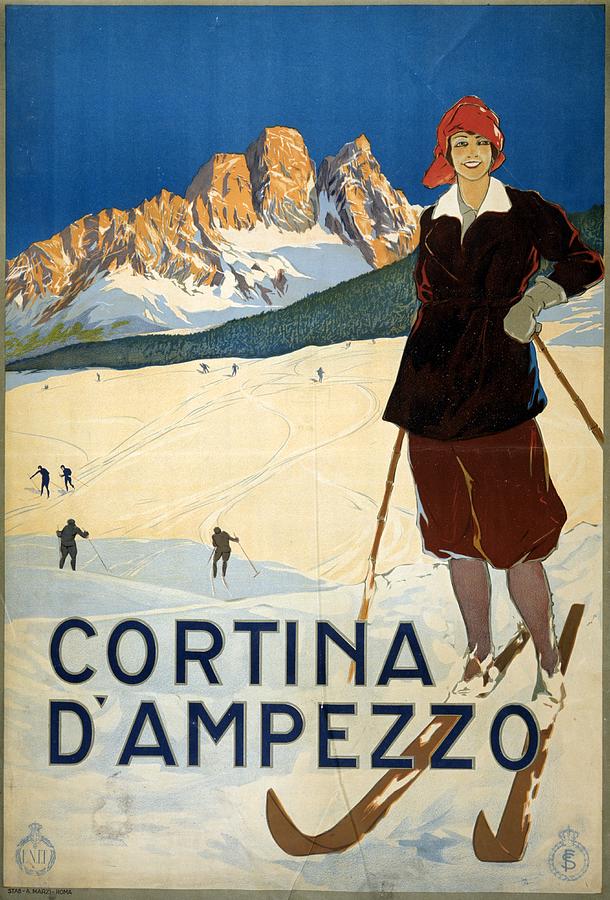This image depicts a vintage skiing poster, prominently featuring a smiling red-haired woman against a scenic, snowy backdrop. The woman, clad in a dark brown short coat, brown knickers or baggy shorts, and a cozy red hat that covers all her hair, stands amidst a picturesque alpine landscape, possibly the Alps. She is equipped with light brown wooden skis that curve up at the tips and holds her ski poles with gloved hands. In the background, rocky beige mountains rise under a shiny, dark blue sky, with other skiers visible in the distance on the snowy hills. Centered on the poster, the text "Cortina d'Ampezzo" is displayed in dark blue or black, suggesting an advertisement for the renowned ski resort. A less legible emblem, resembling a fleur-de-lis, appears in the bottom left corner, further enhancing the poster's vintage charm.